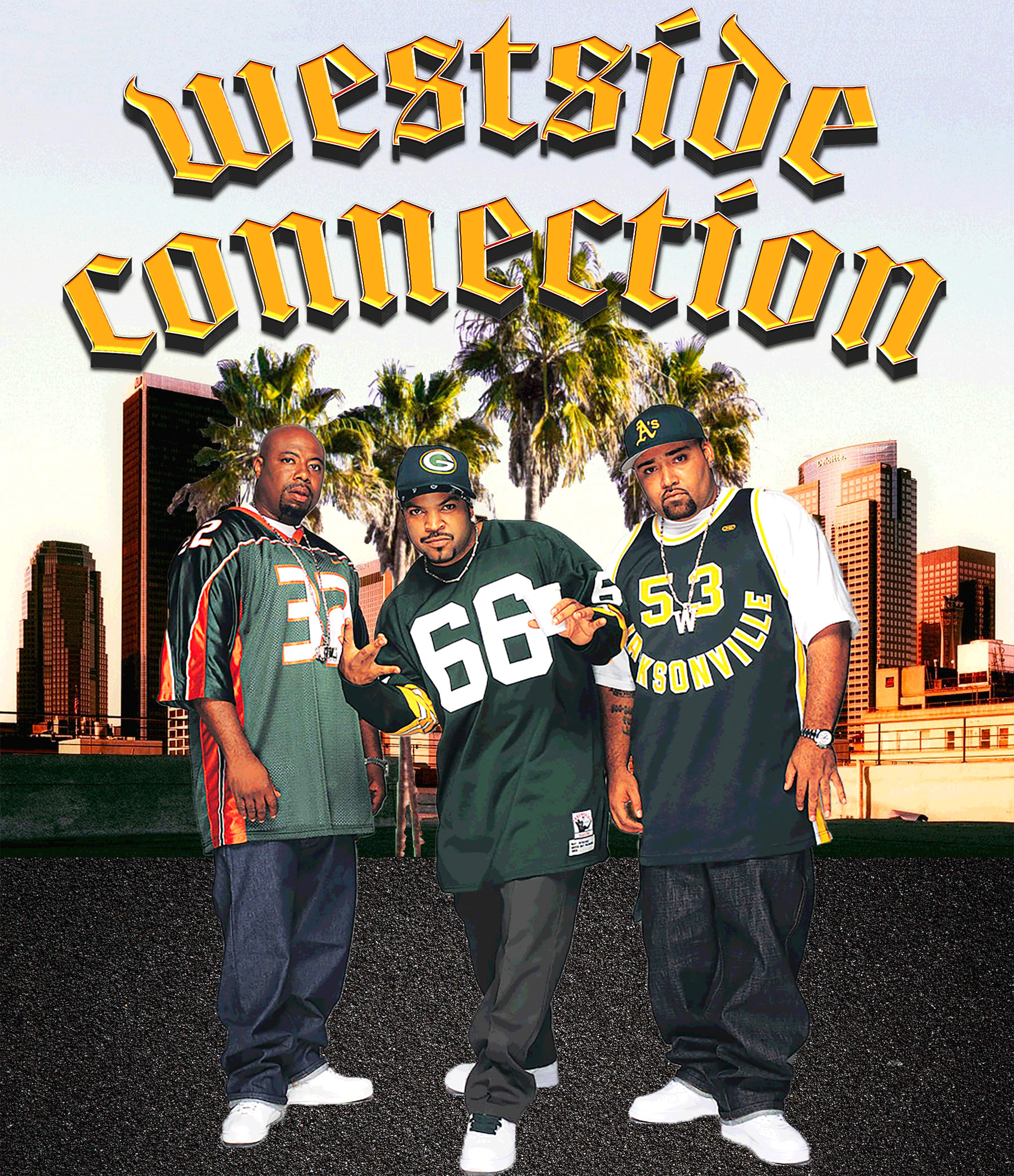This image depicts three men standing on what appears to be an asphalt rooftop with the Los Angeles skyline and palm trees in the background. They are all dressed in sports jerseys and dark pants. The man in the middle, identified as rapper Ice Cube, wears a green jersey marked with the number 66, paired with black pants and white sneakers. He appears to be stepping forward with his left leg and holding a cup in his left hand, while his right hand is gesturing with two fingers pointing toward his body. He also sports a cap and a mustache with heavy gold chains around his neck. To Ice Cube's left, a bald man stands facing slightly to the right, wearing a light green jersey with the number 32, which features dark green sleeves with orange stripes. He complements his outfit with blue jeans and white sneakers. The man on the right is adorned in a green Oakland A's cap with a yellow 'A' and has a bit of a beard and mustache. His blue tank top jersey, numbered 53 and labeled 'Jacksonville,' is worn over a short-sleeved white shirt, paired with blue jeans and white sneakers. He also sports a chain with a pendant that hangs just below the number on his jersey and has a watch on his left wrist. Above them, in prominent yellow letters, the words "Westside Connection" are emblazoned at the top of this vertical, rectangular image.